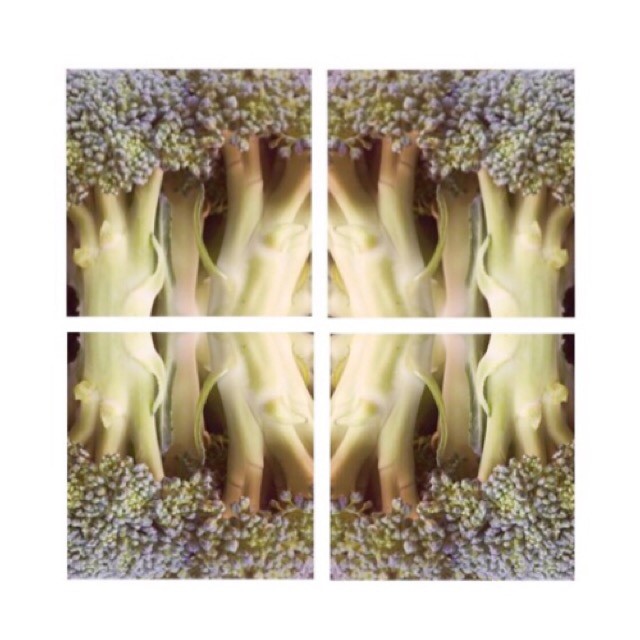The image showcases a meticulously designed arrangement featuring broccoli, divided into a symmetrical design composed of four sections. Each section, an inverted and mirrored version of the others, creates a captivating pattern. The broccoli stems appear light green with a purplish hue transitioning into darker green florets that resemble the tops of trees. The sections are illuminated brightly, highlighting the intricate details. A prominent white cross intersects the image both vertically and horizontally, creating a visually appealing separation. The center of each section features an ovular-shaped, bright white area, contributing to the overall symmetry and tunnel-like effect. The overall presentation of the broccoli gives it a unique, almost artistic appearance, making it a standout piece.